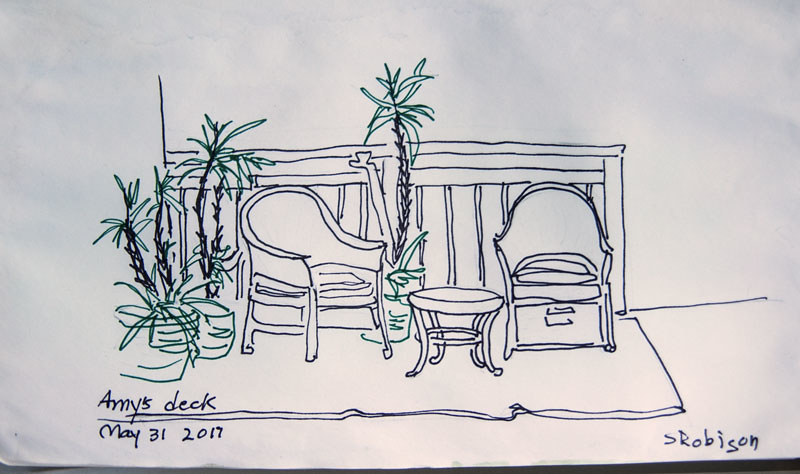This is a highly detailed sketch titled "Amy's Deck," crafted by Robinson and dated May 31st, 2017. The drawing, executed on white paper that might be cardstock, sketchbook paper, or newsprint, utilizes fine tip markers or pens in both black and dark green. The artist employs a nearly continuous line technique, seamlessly transitioning between elements, such as the chairs and the rug they rest on.

The deck scene is framed by a railing and supported by visible posts. Dominating the left side are several potted plants, likely tropical varieties such as banana plants or bamboo, characterized by tall stems and green fronds. These pots, distinctly outlined in dark green, add a lush aesthetic. Two chairs form the focal point, positioned alongside a small round table. The meticulous attention to detail and color contrast between the black lines and green accents enhances the visual depth and realism of the deck scene.